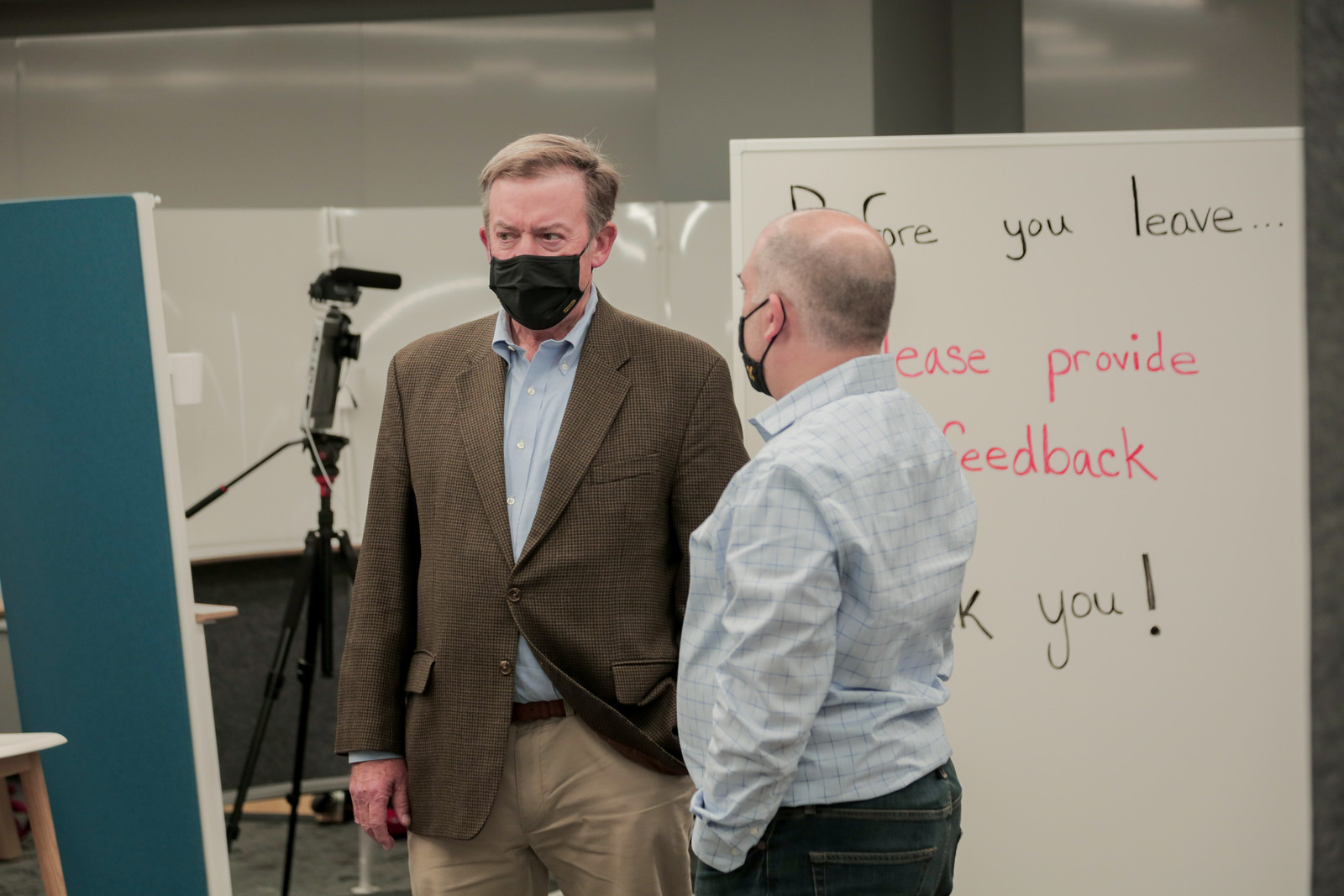The image depicts two men standing and conversing in what appears to be an official or event-related setting, likely from the COVID era given their black face masks. The man on the left, who appears to be in his late 40s or early 50s, wears a brown suit jacket over a blue button-up shirt and khaki pants. He has graying brown hair that is slightly balding. The man on the right, also of a similar age, is bald with short-cropped white hair and is dressed in a light blue checkered button-down shirt and jeans. They stand near a whiteboard with a handwritten sign that reads, "Before you leave, please provide feedback. Thank you." In the background, there is a peculiar flat and tall camera equipped with a boom microphone, positioned inside a booth partitioned by blue and white panels. The setting suggests a conference area or recording studio, indicated by the presence of whiteboards, a stool, and additional recording equipment.